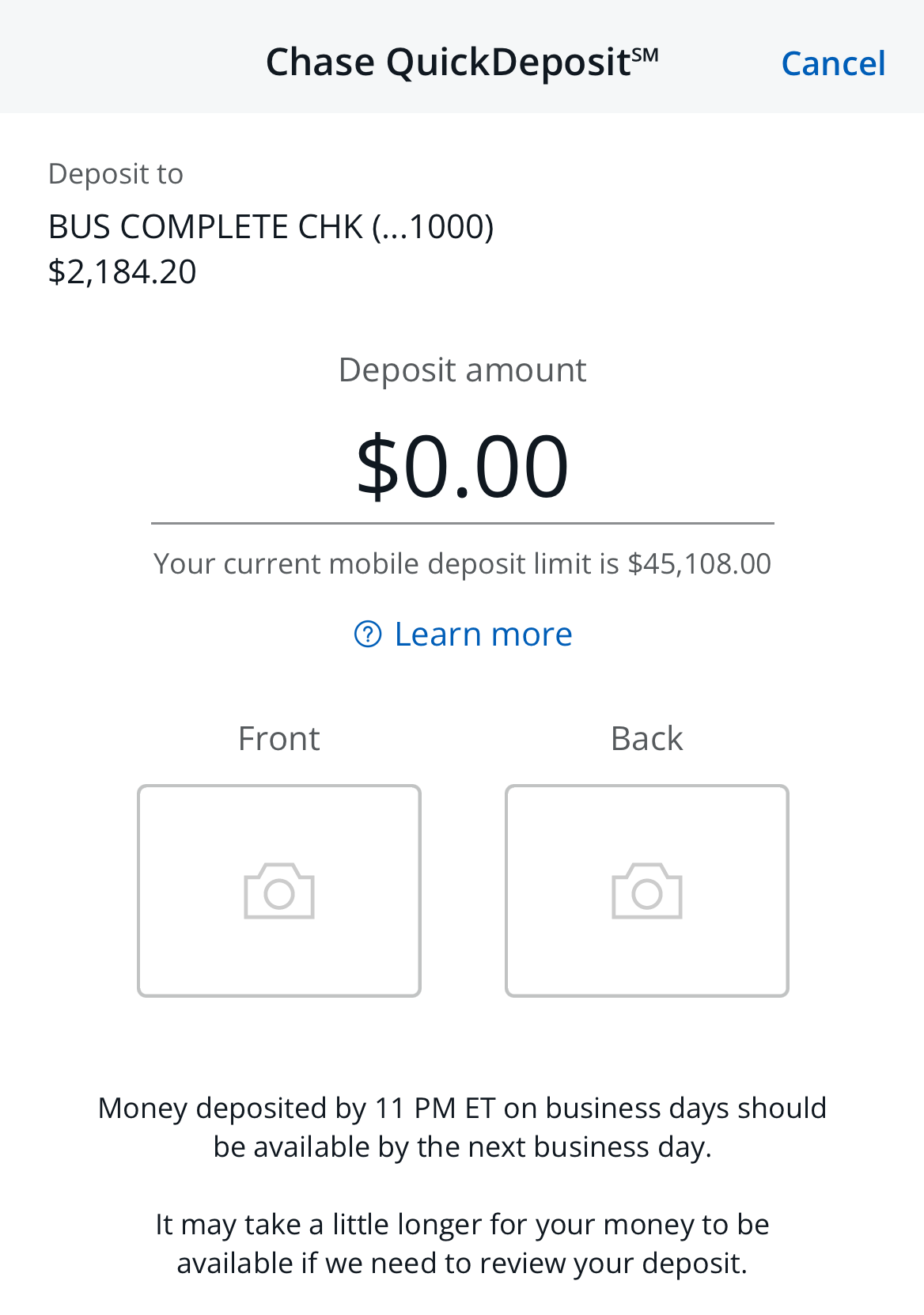In this image, we see the user interface of a bank application, specifically the deposit screen for Chase QuickDeposit. At the top, the header is displayed in a gray box with the text "Chase QuickDeposit." Below the header, the interface shows the deposit account labeled as "Deposit to: Bus Complete CHK," likely indicating a business checking account ending in ...1000.

Directly below the account information, there is a prominently displayed dollar amount, "$2,184.20," which may represent a recent deposit or the account balance. In small gray font, the label "Deposit Amount" appears, followed by a placeholder of "0.00" where users can enter the deposit amount. Beneath this, there is a notification stating, "Your current mobile deposit limit is $45,108."

Further down the screen, there is a "Learn More" option, likely offering additional information about mobile deposits. The interface then shows options for taking photos of the check, with camera icons labeled "Front" on the left and "Back" on the right. Below these options, a message informs users that money deposited by 11 p.m. ET on a business day should be available by the next business day, though availability may be delayed if the deposit requires further review.